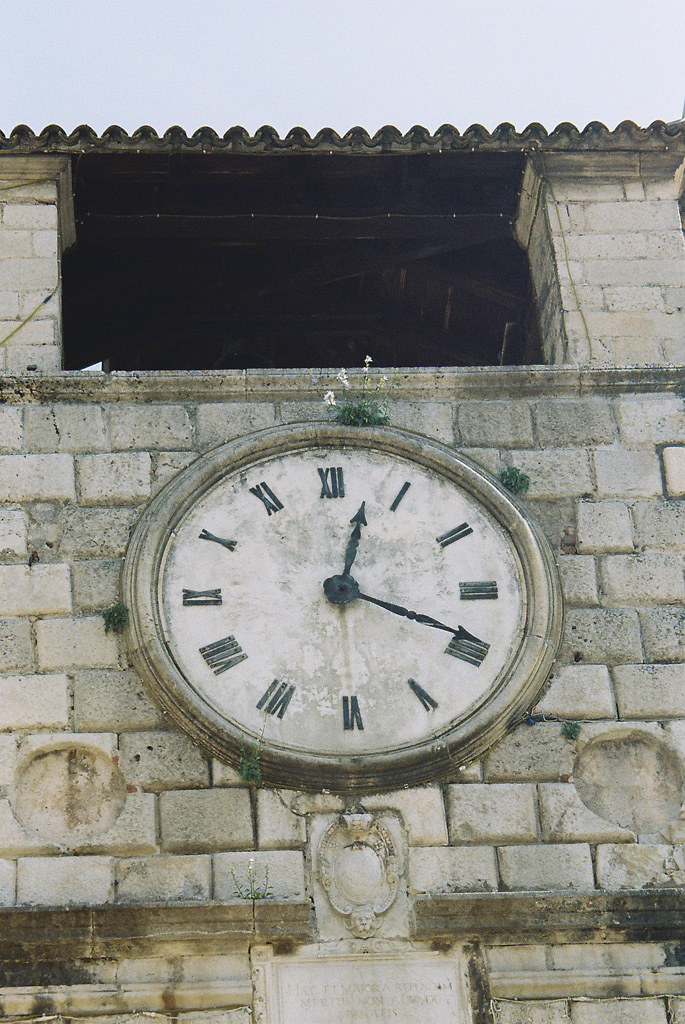This photo is a close-up looking upward at a weathered stone tower or building featuring a prominent, large clock integrated into the façade. The structure itself is made of rectangular, whitish-gray stones. The clock, centered within a circular gray stone border, has a dirty white face displaying Roman numerals from I to XII. Both the hour and minute hands are black, showing the time as 12:19. Above the clock, two square columns frame a rectangular opening with a dark background, which may lead into a belfry. The roof above this opening has a distinct, swirly design. Below the clock, there is a medallion and a plaque with unreadable lettering. The entire scene evokes a sense of historical architecture with its weathered materials and classic design elements.